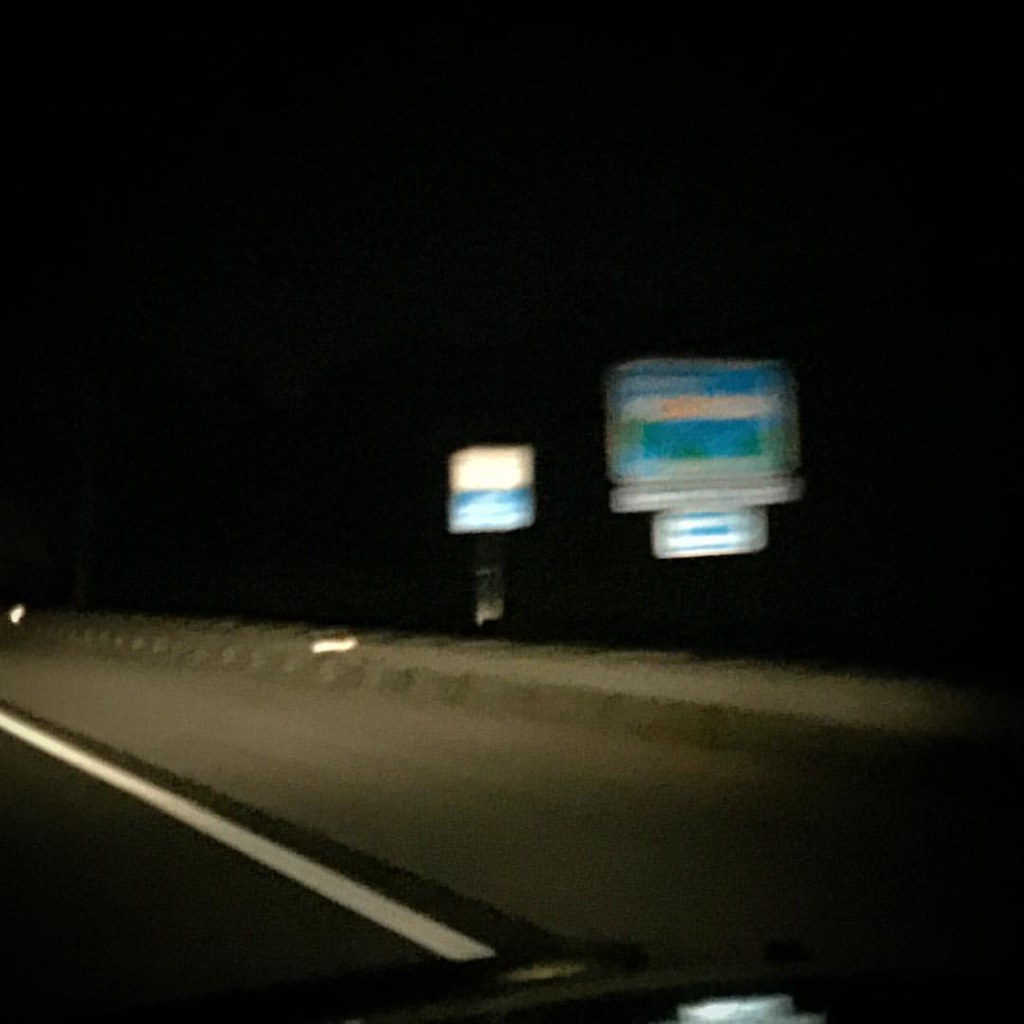The image is a very blurry nighttime photograph taken from a moving car. The sky is pitch black, and the road is dimly visible with a white line running along its edge. The road transitions from gray to brown, suggesting a shoulder or different lane, and there's a curb with the ground slightly elevated beyond it. The lower left part of the image shows the road, while the right side transitions from brownish dirt to greenish tones and then becomes black towards the corner.

Two highway signs are blurry and reflecting light. The larger sign on the right is mostly a blue rectangle with light blue, green, orange, and white elements. Below it, a smaller gray-outlined rectangle contains white and blue stripes. Another sign to the left has an orange top section and a blue bottom. Additionally, there is a glowing white object near the curb, possibly a reflective marker.